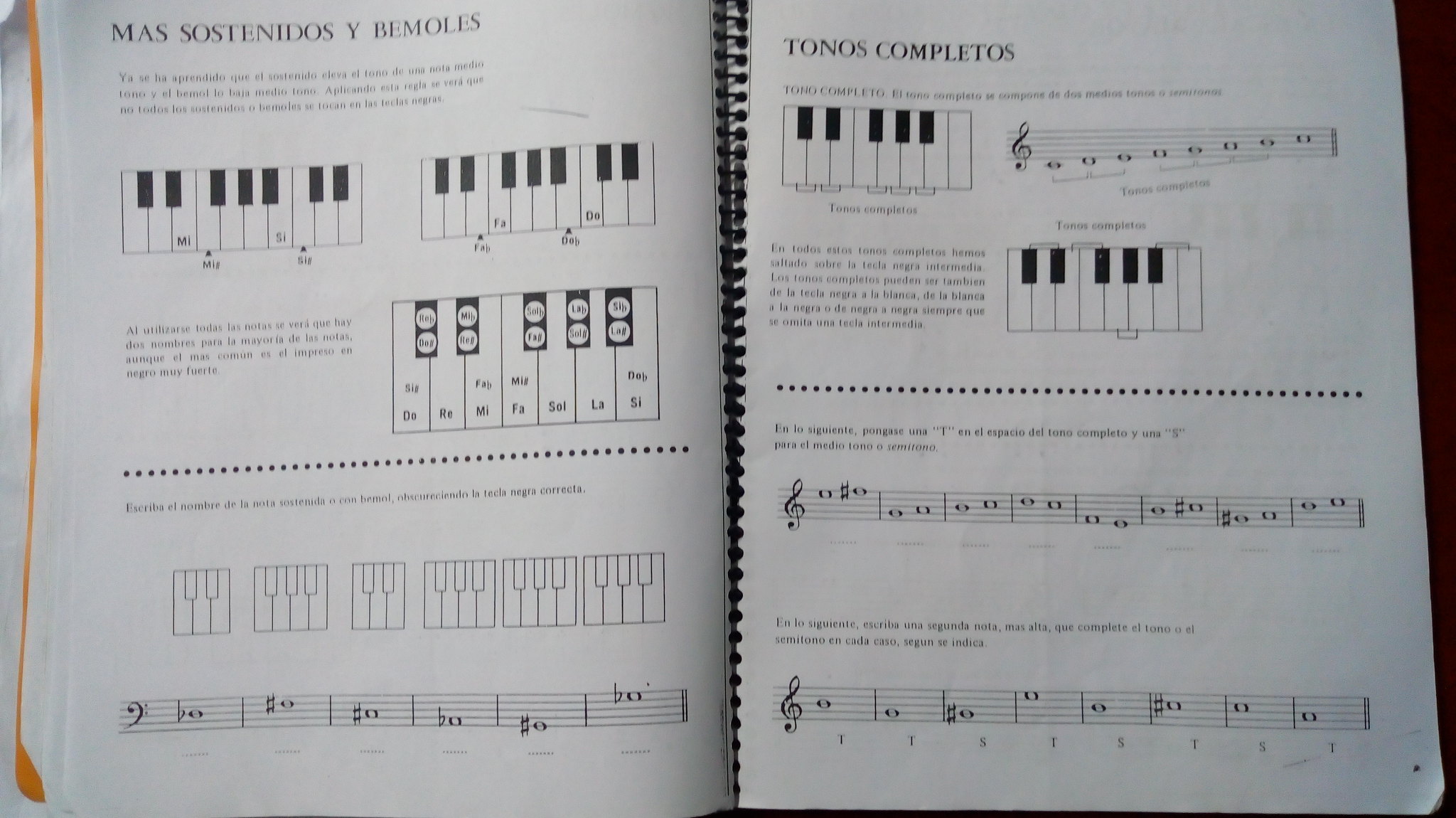This is a detailed photograph of two pages from a piano instruction manual, written in Spanish, that lays open on a desk. The pages are part of a spiral-bound book, with white pages and black text and graphics. On the left page, the heading reads "Mas Sostenidos y Bemoles" and features a top-down view of piano keys labeled with letters. The right page is titled "Tonos Completos" and includes another image of piano keys, along with a snippet of sheet music. Below the heading, there are two lines of sheet music accompanied by additional Spanish text. The graphics and text are all in black and white, making up the primary focus of the photograph.